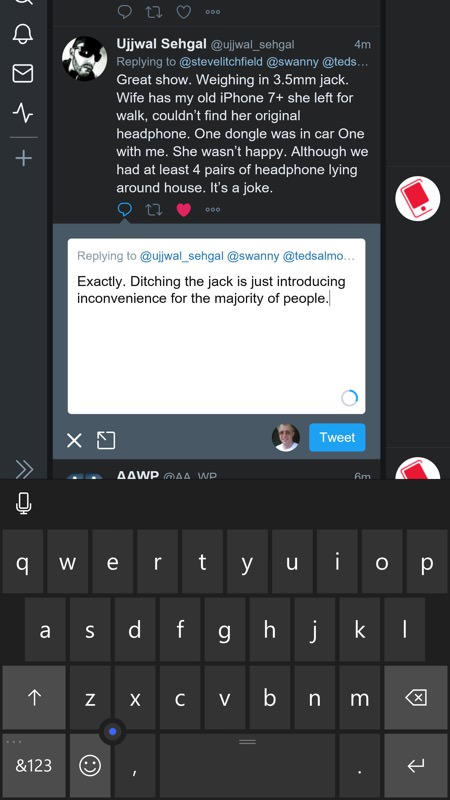This is a screenshot of a smartphone display showing a social media interaction on the platform formerly known as Twitter, now called X. The interface includes a left sidebar with various icons: a bell, an envelope, a plus sign, and a sideways Z. 

The main content is a tweet from a user with the handle Ujjwal Sehgal, whose profile features an animated image of a white man with black hair, a black mustache, a black beard, and dark sunglasses. Ujjwal is responding to a discussion initiated by Steve Litchfield, who is tagged along with other users. The tweet reads as follows:
"Great show, weighing in on the 3.5mm jack. Wife has my old iPhone 7 Plus; she left for a walk and couldn't find her original headphones. One dongle was in the car, and one was with me. She wasn't happy, although we had at least four pairs of headphones lying around the house (typo on 'headphones')."

Following Ujjwal's tweet is a reply criticizing the removal of the headphone jack, stating, "Ditching the jack is just introducing inconvenience for the majority of people," accompanied by another user's profile icon—a white man with glasses and short hair, wearing a white shirt.

The right side of the screen features a "Tweet" button in a blue box. Below the interface, the phone's typewriter-style keyboard is visible. The device itself is white with red accents, including two circular elements on the right edge of the phone's frame.